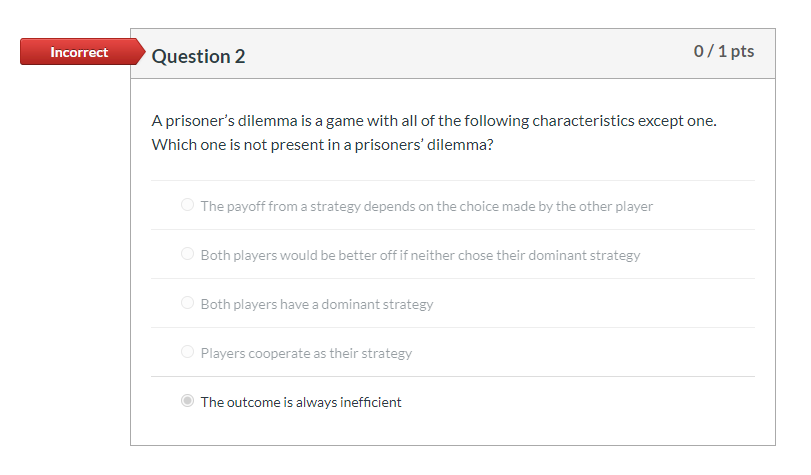Screenshot of a multiple-choice question in an assessment, marked incorrect. The interface features a one-pixel outlined header with a white field below displaying the question and options. Adjacent to the question, a red rectangle with a triangular edge points to it, with "Incorrect" written in white text inside the red shape. To the right, it indicates "Question 2, 0 of 1 points."

The question reads: "A prisoner's dilemma is a game with all the following characteristics except one. Which is not present in the prisoner's dilemma?" There are five options listed in gray text, except the selected one, which is highlighted with a radio button. The options are:

1. The payoff from a strategy depends on the choice made by the player.
2. Both players will be better off if neither chose their dominant strategy.
3. Both players have a dominant strategy.
4. Players cooperate as part of their strategy.
5. The outcome is always inefficient (selected and marked incorrect).

The correct answer is option 2: "Both players will be better off if neither chose their dominant strategy." The overall design is minimalistic with a plain white background and no additional elements.